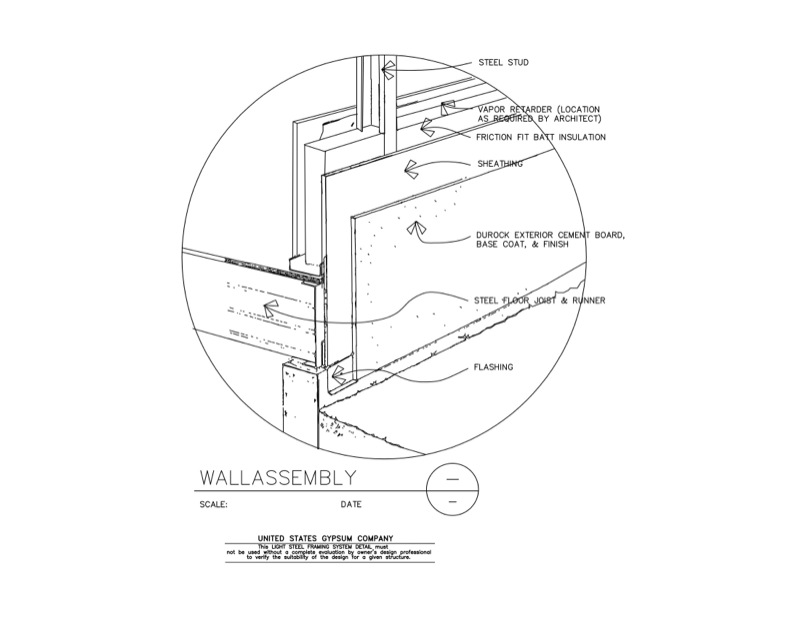This image is a detailed schematic illustration of a wall assembly, labeled as such beneath the diagram. The depicted wall assembly is enclosed within a perfect circle and carefully details each layer of construction with corresponding labels and arrows pointing to specific elements. The labels list the following components, starting from the innermost layer going outward: steel studs arranged vertically, followed by a vapor retarder whose placement is specified by an architect, and friction-fit bat insulation. The diagram also includes sheathing, Duroc exterior cement board, and subsequent base coat and finish, indicating paint. Additionally, it delineates a steel floor and joint runner arranged parallel to the layers, and finalizes with flashing at the bottom, which completes the framed wall or corner. At the bottom of the image, "United States Gypsum Company" is written, along with placeholders for scale and date, though these details are not filled in. The schematic is rendered in black and white and features textural details for clarity.